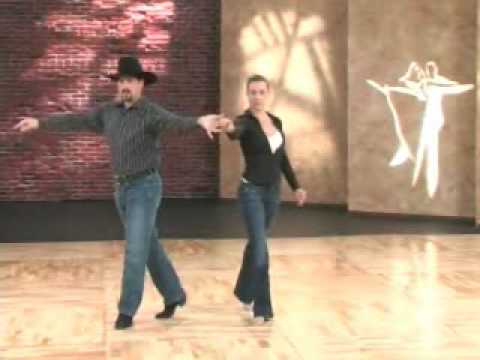In this grainy photograph capturing a dynamic moment from a dance routine, a couple dressed in Western attire is seen performing. The man on the left, wearing a black cowboy hat, green striped button-up shirt, blue jeans, and cowboy boots, extends his arms to his sides. The woman beside him, holding his hand, is dressed in flared bell-bottom jeans and a black long-sleeve shirt over a white tank top. They dance on a gleaming parquet wooden floor that contrasts with the black flooring towards the back. The backdrop features a mix of a red brick wall and two tan-colored panels, with light streaming through a window onto one of them. A silhouette of a dancing couple is prominently displayed on one of the tan panels, enhancing the lively, dance-focused ambiance of the scene.